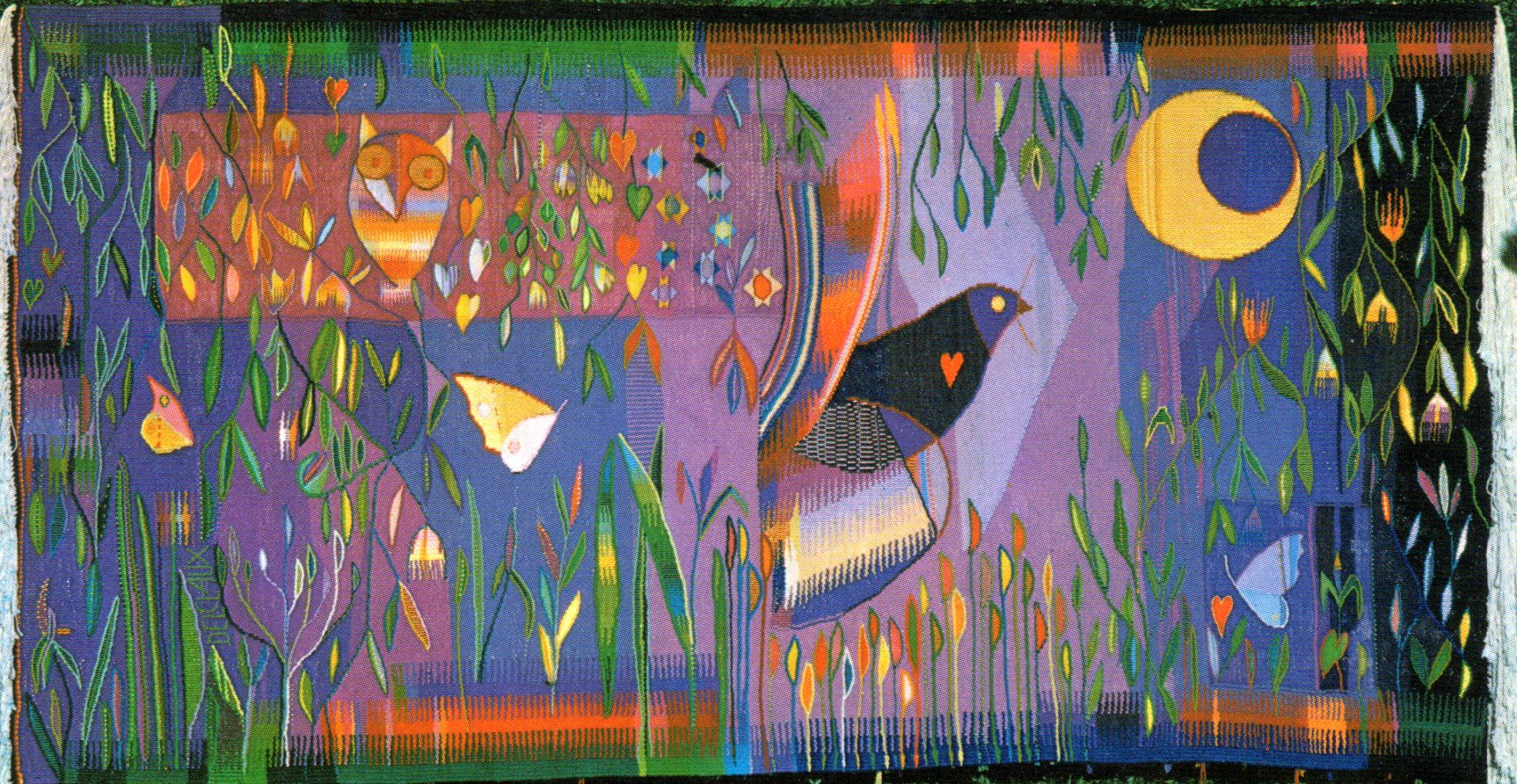This vibrant, multi-colored artwork, possibly a painting or tapestry, features a dynamic and detailed composition. Dominating the center of the piece is a striking bird with a blue head, black body, and a red heart prominently displayed on its side. The bird holds a twig in its beak and stands against a blue background. To the right of the bird is a uniquely shaped crescent moon, which almost resembles a full moon where the top and bottom of the crescent touch. Below this are two butterflies, with at least one in a light blue hue tinged with darker blue, flying across the image.

In the bottom-left section of the artwork, among twigs and leaves in various shades of green, yellow, and orange, sits an owl. The owl, marked by its pointy ears, nose, and bug eyes, has a teardrop-shaped body and is placed against an area marked off in brown. Towards the left side, the background is more of a blue hue transitioning into purple and pink toward the right, with green vertical lines and a vine with elongated leaves.

The painting also includes other butterflies, some in orange and white, enhancing the overall vibrant and lively atmosphere. The edges of the piece look slightly raveled or worn, adding to the tapestry-like feel of the artwork.